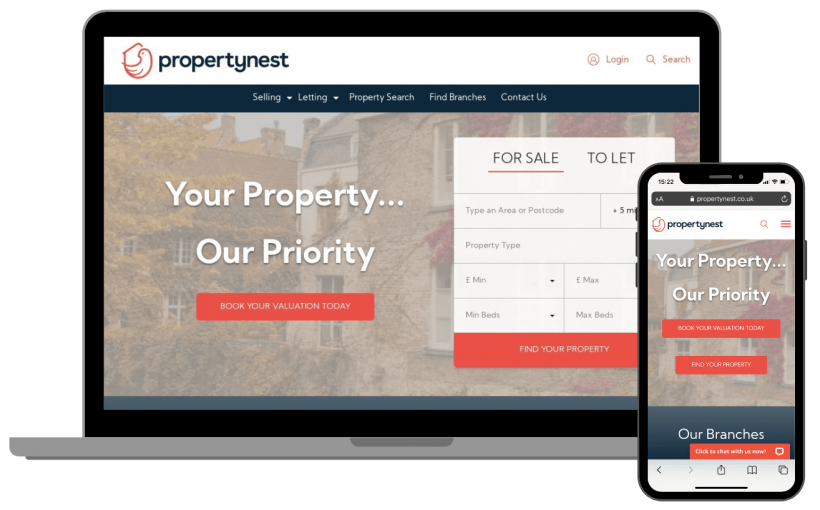A screenshot from a property website is displayed, showcasing its layout on both a laptop and a mobile phone. 

On the laptop interface, we observe the bottom half of a gray laptop screen, bordered by a black band, without visible keys. The screen exhibits a mock-up of the website, designed to demonstrate its appearance on different devices. At the top of the laptop screen, a white banner prominently features the website's logo on the left—depicting "Property Nest" in dark blue text beside an abstract hand or bird icon holding a piece of paper, outlined in red. To the right of the logo are clickable options for "Login" in red and a "Search" icon. Beneath the white banner is a dark blue navigation bar with categories such as "Selling," "Letting," and "Property Search," although the remaining labels are too small to decipher. Below this, a background image of trees and buildings is overlaid with the slogan "Your Property, Our Priority" in white text. An orange box beneath this banner contains small, unreadable text, leading down to a section on the right where users can choose between "For Sale" or "To Let" options, and fill out accompanying fields, ending with another orange button.

The mobile version mirrors the desktop site in design. Positioned at the top is a black search bar, followed by the property website's logo and white bar. The familiar background image with the "Your Property, Our Priority" slogan is present, succeeded by two orange boxes with white text. The section marked "Our Branches" appears below in blue with white text, followed by another slightly right-tilted orange box. The interface concludes at the bottom with visible mobile phone keys.

The detailed screenshot provides a clear understanding of the website’s adaptive design across devices, emphasizing user accessibility and consistent branding elements.